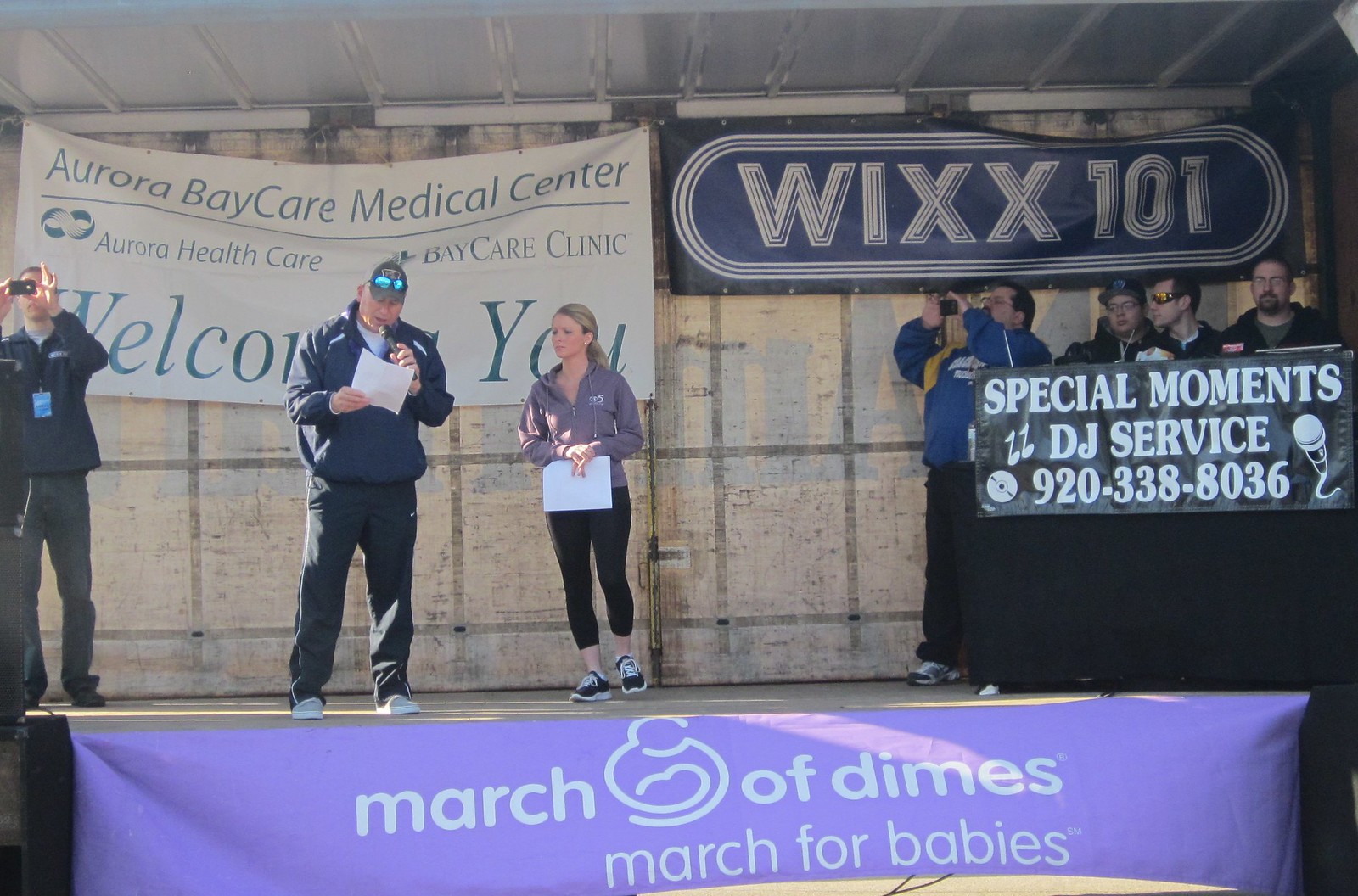The image captures a lively event set on a stage adorned with various banners and logos. Central to the scene is a sign that reads "March of Dimes, March for Babies" in purple with white font, indicating a charity event. On stage, a diverse group of seven people are prominently featured. A woman with blonde hair pulled back, dressed in a purple sweater and black leggings, stands beside an older man clad in a blue tracksuit and a baseball cap with sunglasses perched on top. He holds a piece of paper and speaks into a microphone, while the woman attentively listens. To their left, another man is seen taking pictures of the audience. In the background, a sign from "Aurora Bay Care Medical Center, Aurora Health Center Bay Care Clinic" extends a warm welcome, alongside another banner for "WIXX101." To the right, several men, visible only from the shoulders up and dressed in dark colors, stand behind a dark podium draped with a banner for "Special Moments DJ Service," complete with contact information and a microphone icon. The stage is bustling with activity, encapsulating the spirit of the event.